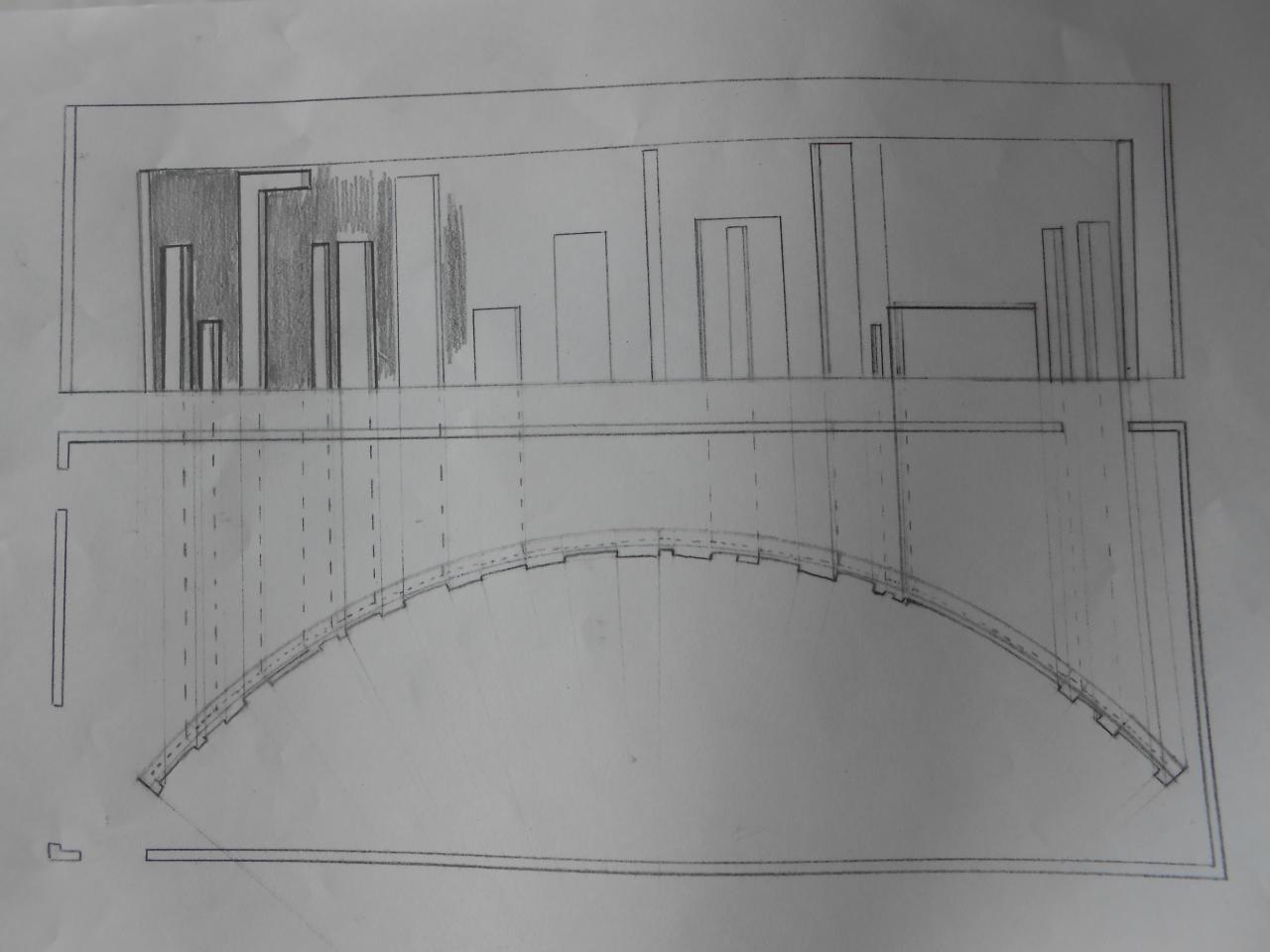The drawing appears on a piece of white printer paper that is slightly wider than it is tall. The sketch is drawn with a pencil and appears unfinished. The bottom section features a roughly drawn rectangular border composed of two lines, within which there's an arched structure resembling a bridge. From this arch, dashed lines extend upwards, leading to the top section of the paper. The upper section contains a series of 3D rectangles of varying sizes arranged like buildings in a skyline. One of these rectangles is uniquely shaped like an upside-down "L." Additionally, the left portion of this top section is partly shaded, with the shading stopping about a third of the way across the drawing. The overall impression is of a conceptual architectural sketch, possibly depicting a bridge leading to a group of buildings.